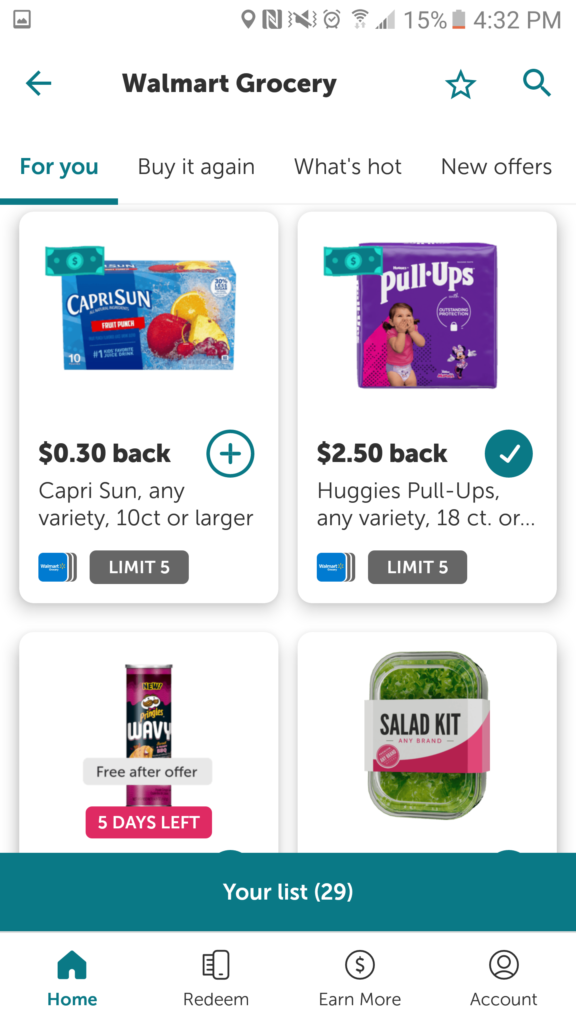The image captures a mobile device displaying an advertisement for Walmart Groceries. At the top of the screen, there's a header labeled "Walmart Groceries," accompanied by an arrow pointing left, a star icon, and a magnifying glass. Various icons such as for picture, navigation, sound, time, Wi-Fi, phone signal, and timer are also visible, indicating the device's status. The battery level is notably low at 15%.

The advertisement showcases four main promotional items arranged in rectangular sections. The first item is a box of Capri Sun, offering a 30-cent cashback on any variety for a 10-count or larger pack, with a limit of five redemptions. Beside it is a promotion for Huggies Pull-Ups, providing a $2.50 cashback on any variety for an 18-count pack, also with a limit of five redemptions, and a checkmark indicates this offer has been activated. Adjacent to this is an advertisement for Wavy Pringles, highlighted with "Free after offer" and a note that the deal expires in five days. The final section advertises a salad kit.

Below these offers, there's a summary listing "Your List" with a total amount of $29. Four icons at the bottom of the screen represent navigation options: "Home," "WeDean," "Earn More," and "Account."